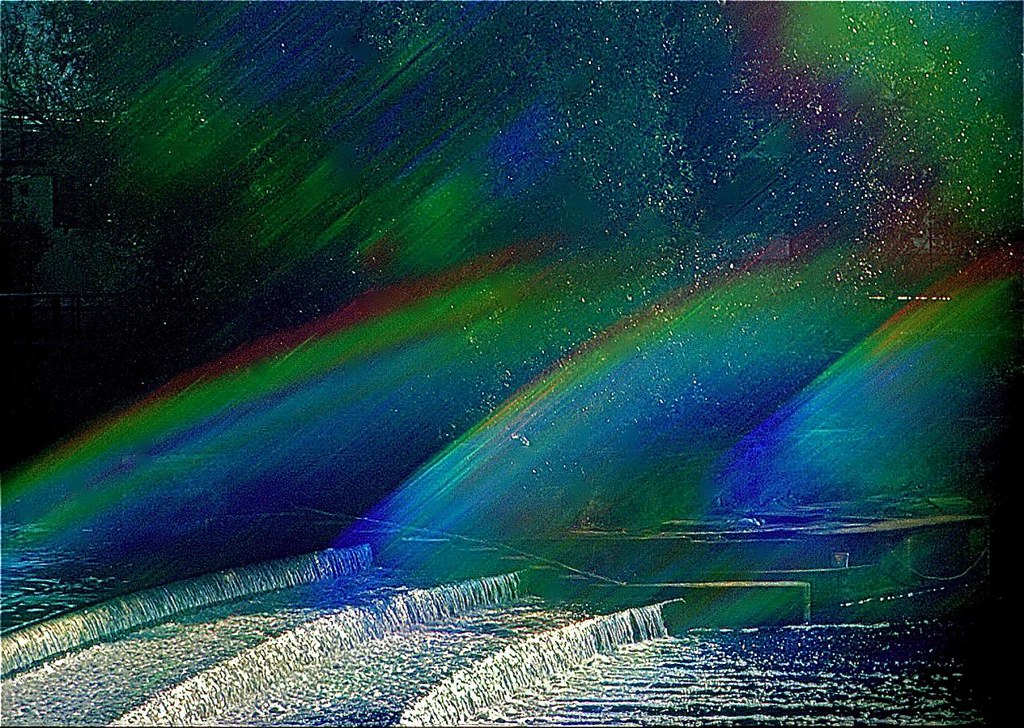The image depicts a vibrant and dynamic scene that combines elements of nature and architecture, seemingly captured in a detailed oil painting with a predominantly gray backdrop. Dominating the canvas is a sequence of three step-down platforms or ridges in a waterway, where water cascades down each level, eventually spilling into a pond below. These platforms, distinctly gray with visible ridges, are depicted with a serene flow of water creating delicate white waves against a darker blue undertone. The waves are highlighted by thin white streaks flowing horizontally, enhancing the sense of movement.

Towards the right side, an indistinct outline of what appears to be a boat or another vague vehicle emerges, adding a hint of human presence. Rising above this scene in the sky, streaks of green, red, and blue cascade down, reminiscent of the ethereal glow of the northern lights. The upper right corner features a green splotch of paint adorned with white dots, evoking the imagery of stars set against a sea-green backdrop, interspersed with shades of purple, blue, and more green leading towards the upper left corner, punctuated by a white splotch.

On the left side of the painting, amidst this vibrant color play, darker shades, almost black, transition into a rainbow of colors — red, yellow, green, and light blue — emanating from the center towards the lower parts of the painting. Nestled above this natural display are what resemble the branches of a tree, and a small building perched on the upper left, overseeing the flowing waterfall area, adds an architectural element to the serene, yet vivid landscape. At the bottom, a delicate footbridge extends, completing the picturesque setting depicted in this richly detailed work of art.